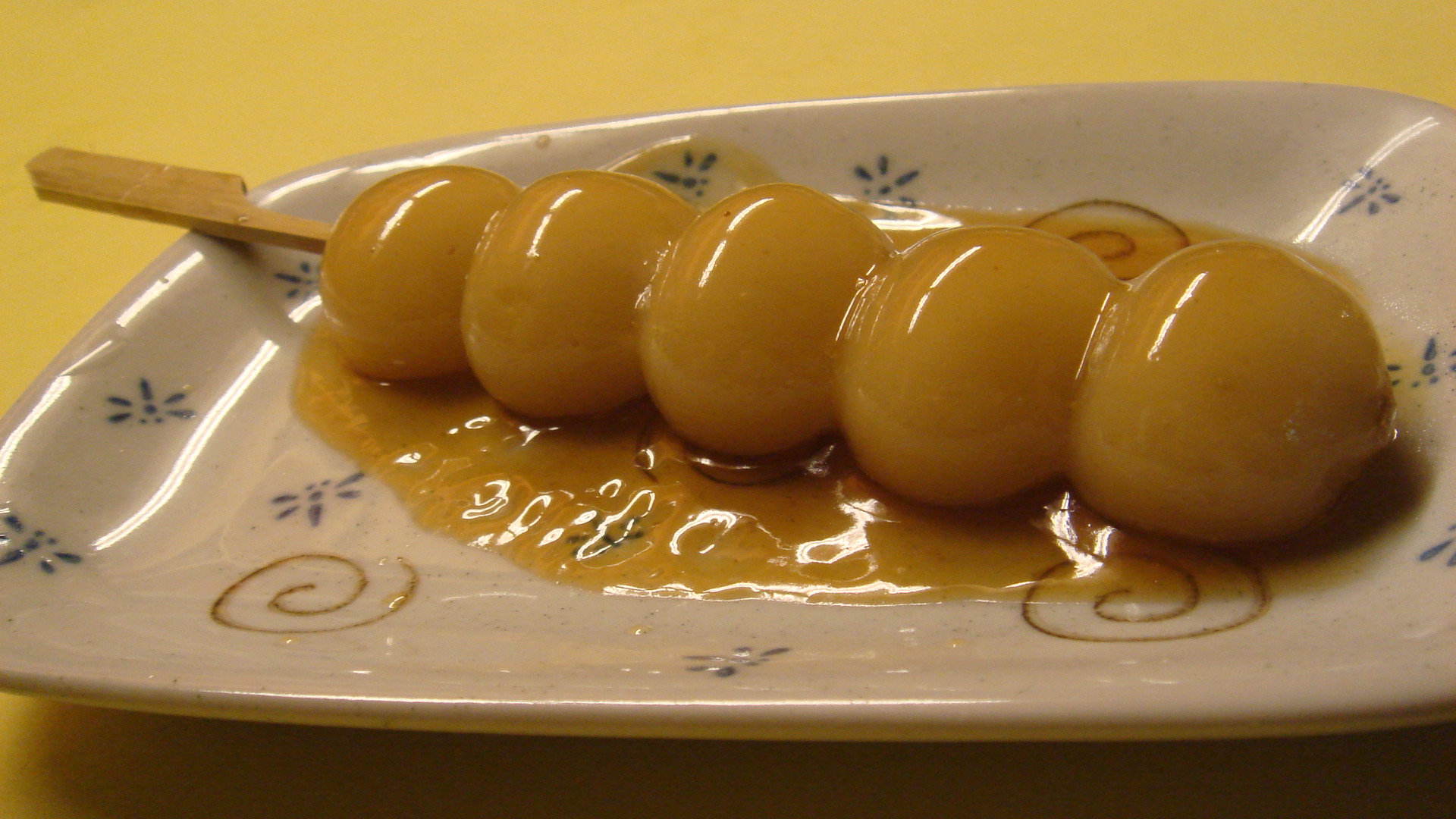The photograph showcases a wooden skewer with five glossy, yolk-like balls arranged on it. The skewer is suspended over a white ceramic plate that features intricate blue floral patterns and red, swirling designs reminiscent of snails. This porcelain plate appears aged yet detailed, contributing to the vintage aesthetic. Below the skewer, a shiny liquid drips into a small dish that mirrors the same delicate blue and red designs. Despite the captivating subject, the image suffers from lack of clarity and focus, making the scene slightly blurred. The backdrop is a mustard yellow, likely a counter or a piece of paper, providing contrast but no additional context or identifying information.